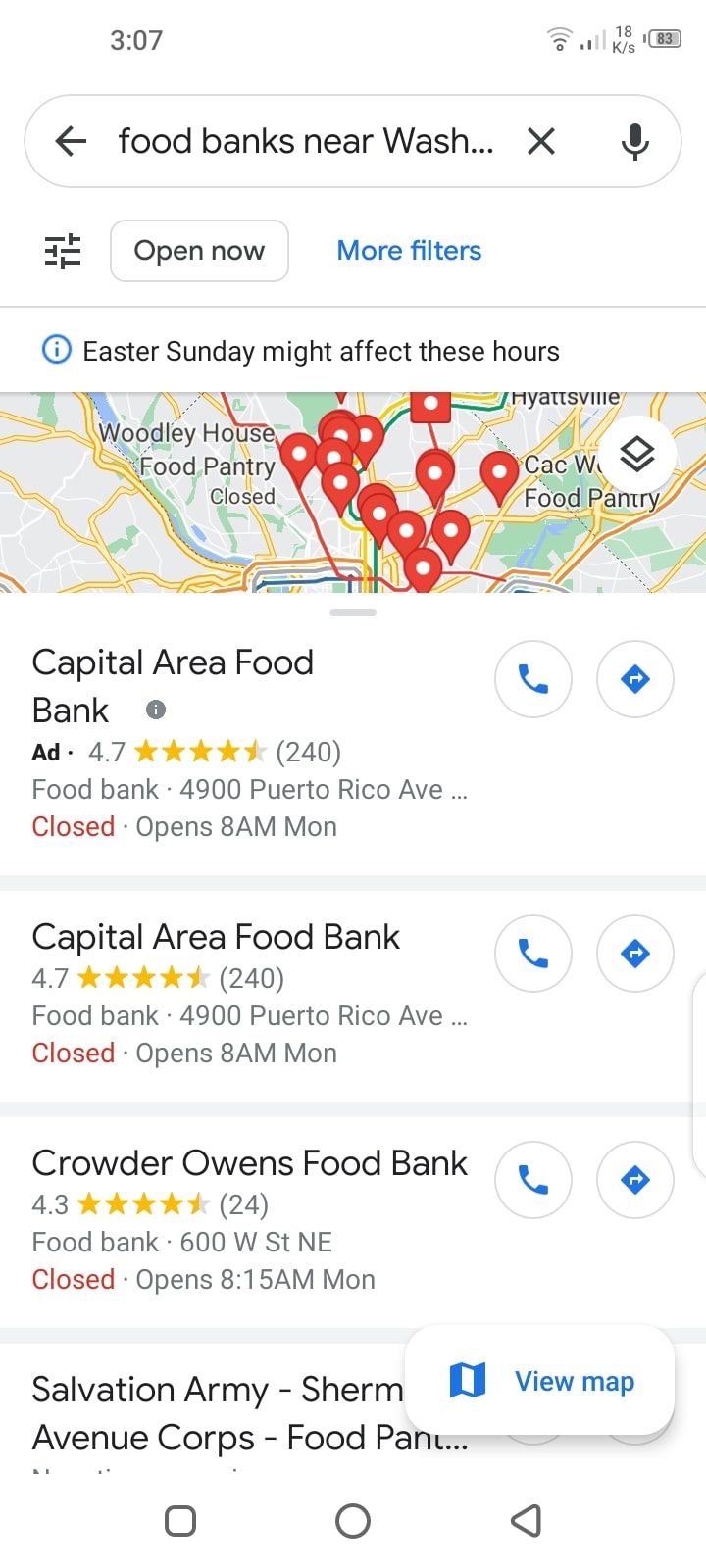The image is a screenshot taken from a smartphone. It captures a search results page with a predominantly white background. At the top of the screen, the status bar displays the time, 3:07, along with the WiFi signal, network signal, and battery icons.

Below the status bar is a search interface. The search bar includes a left-pointing black arrow, incomplete text reading "food banks near wash...", a 'X' button for clearing the search, and a microphone icon for voice search. Below the search bar, there are interactive elements such as a 'Filter' button, an 'Open Now' filter option, and a 'More Filters' link highlighted in blue.

There is a cautionary note in black text mentioning that Easter Sunday might affect the service hours. Following this, a map is displayed showing multiple locations with red and white location pins.

Below the map, the search results list food banks along with their relevant details. The first listed is the "Capital Area Food Bank," showing its ratings with yellow stars, and its status as "Closed," indicated in red. The address is also provided, along with clickable options to call the food bank or get directions. Another listed location is "Crowder Owners Food Bank," which is also marked as "Closed." Similar options for calling and directions are provided for each entry.